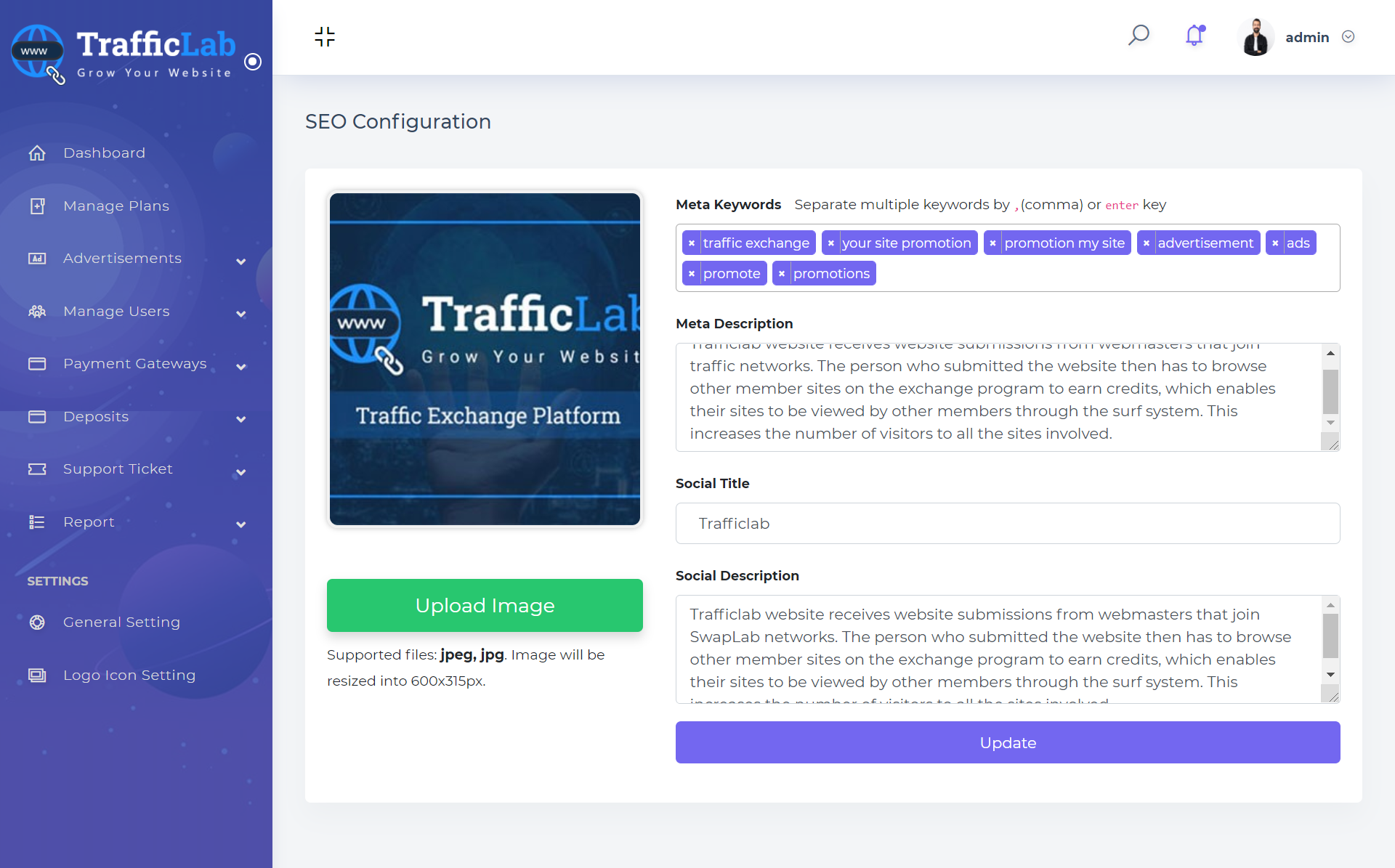The image appears to be a screenshot of a web page dedicated to traffic information management. On the left side, there's a vertical column in a purplish-blue color featuring approximately 10 clickable options. The bottom two options are labeled "General Settings" and "Logo Icon Settings." 

Adjacent to this column, on the right, there's a larger white rectangular section. At the top-right corner of this section, there are three elements: a magnifying glass icon, a notification bell icon, and a label saying "Admin" accompanied by a profile picture. 

In the main white rectangular section, there's a prominent black square displaying the text "Traffic Lab, Grow Your Web Site" – however, the "E" in "Site" is missing – followed by the text "Traffic Exchange Platform." Below this, there's a green rectangle titled "Upload Image," indicating that supported files are JPEG and JPG, which will be resized to dimensions of 600 x 315 pixels.

Further down, there are additional sections titled "Meta Keywords," "Meta Description," "Social Title," and "Social Description." Beside these sections, there is a bar featuring two options, one of which is for updating the information.